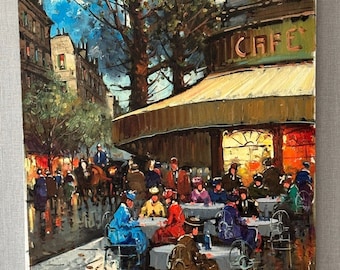The image is a small, impressionistic painting depicting a bustling outdoor café on the corner of a crowded downtown street in an old city, possibly Paris, from the late 19th or early 20th century. The café, with its yellowish-brown awning and green sign reading "café," features tables and chairs filled with people dressed in formal Sunday attire typical of the era, with women in bulky dresses and round hats. The street is lively, with numerous pedestrians, a policeman on horseback, and a horse and buggy. Trees are scattered around, and the sky is a deep blue with patches of clouds. The buildings in the background are multi-story and closely spaced, adding to the intimate, urban feel. The painting’s impressionistic style renders the scene dreamlike and hazy, with vibrant colors and inviting details, though the faces of the people remain undetailed.